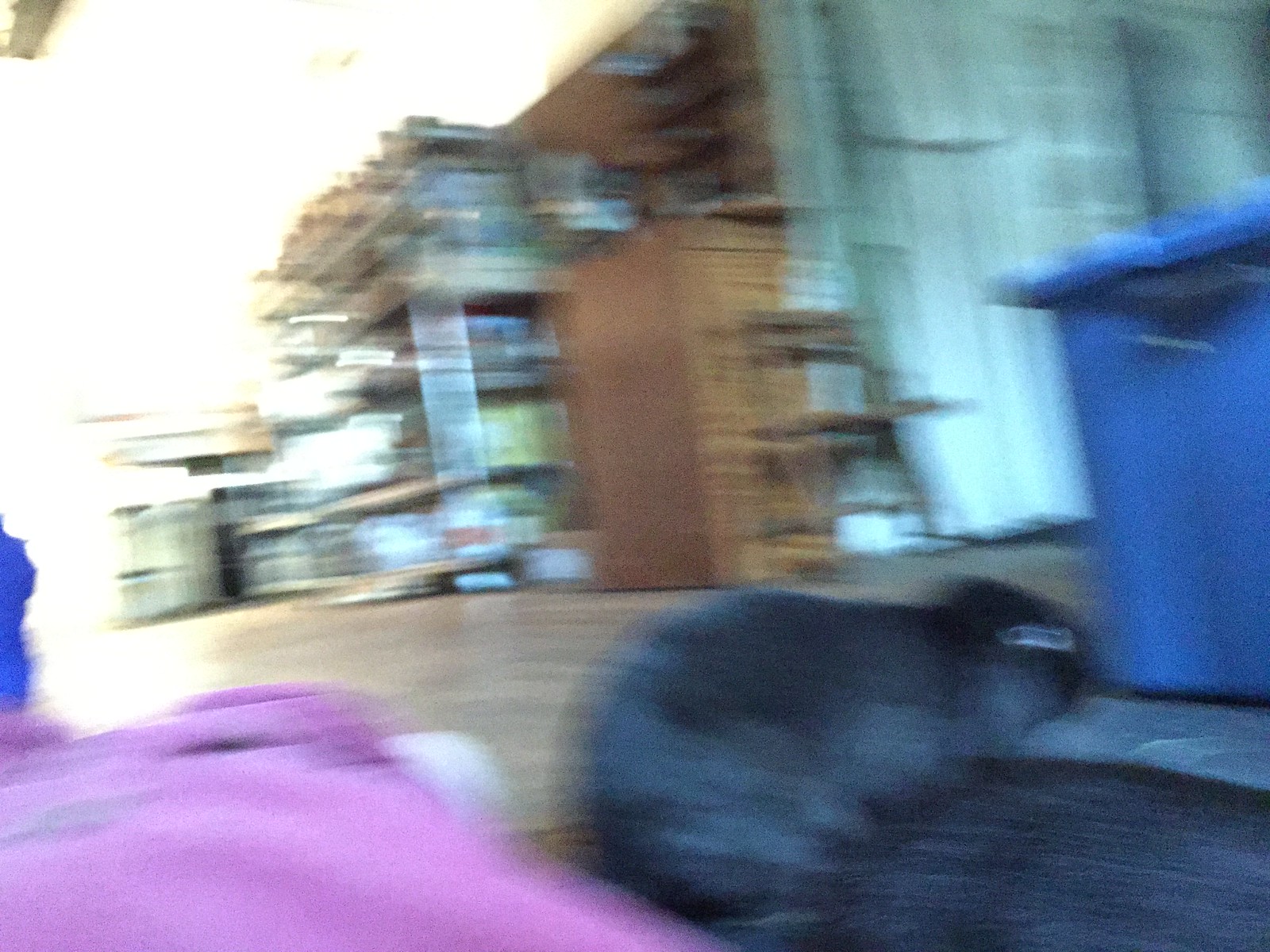The blurred image depicts an outdoor or back alley setting. To the right, there is a large blue trash can resembling a dumpster. In front of this, the camera captures two items: one is purple and the other is black, possibly fabric material or pillows. Centered in the foreground, there is a sizeable piece of brown wooden furniture, either a table flipped on its side or a cabinet/dresser. Adjacent to this wooden piece, a shelf can also be seen.